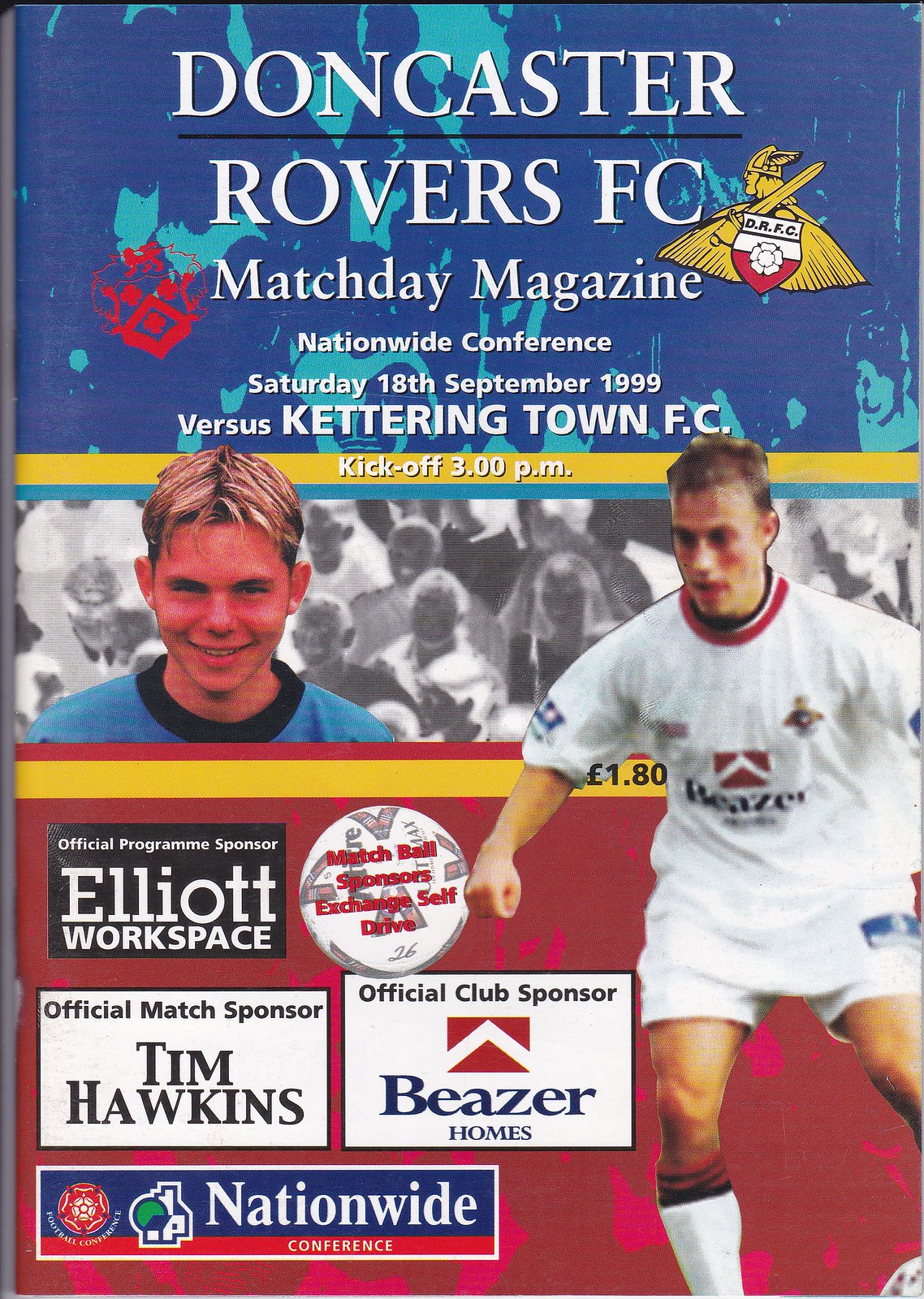The cover of the Doncaster Rovers FC Match Day Magazine for the Nationwide Conference, dated Saturday, 18th September 1999, features a vibrant blue banner at the top with white text stating the event details and a yellow strip indicating the 3pm kickoff time. Prominently displayed is the team logo, depicting a Viking with a flowing cape, holding a sword on his shoulder and wearing a winged helmet. The Viking's shield bears the DRRC initials, split into red and white halves.

The bottom section of the cover showcases two images: a headshot of a young player in a blue shirt, set against a background of an inverted black-and-white crowd, and a full-body image of another player in mid-kick, although the rough cutout makes this image less seamless. At the very bottom left, several sponsor logos are visible, including Elliott Workspace, Nationwide Conference, Tim Hawkins, and Reaser Homes. The program is priced at £1.80.